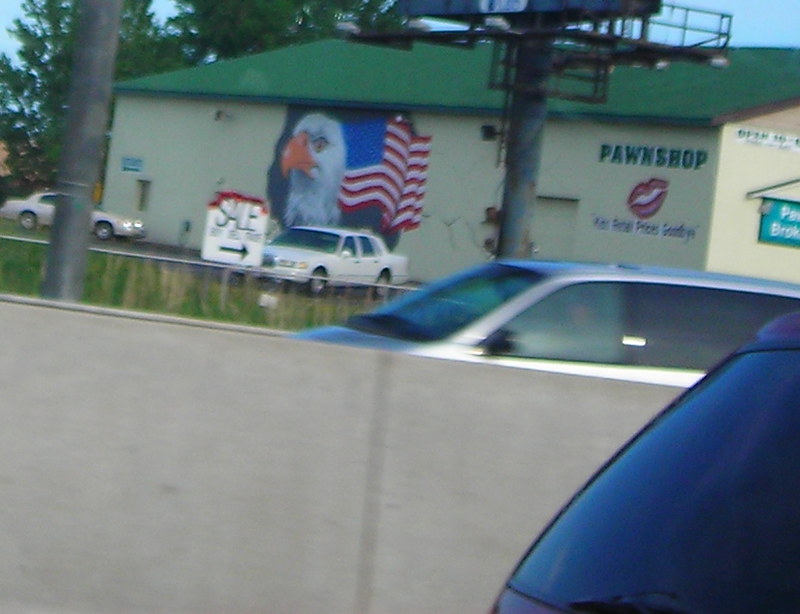The image depicts the side of a large building, identified as a pawn shop. The structure features a striking mural showcasing the head of a bald eagle with a piercing yellow eye and an orange beak, set against a yellow background. Behind the eagle, an American flag appears to be blowing in the breeze, complete with its iconic blue corner adorned with white stars and red and white stripes. The roof of the building is a prominent dark green, while the walls are a tan or yellow color. On the right side of the building, there is the sign "pawn shop" in green text over a stylized pair of red lips, under which the phrase "kiss retail prices goodbye" can be seen. In front of the building, there is a sign pointing to the pawn shop with the word "SAIL." The scene includes a silver minivan and another car in the divided lanes of the road ahead, separated by a long wall. Two vehicles are parked directly outside the pawn shop, while the lower part of a billboard, complete with its pole, ladder, and scaffolding, stands nearby.